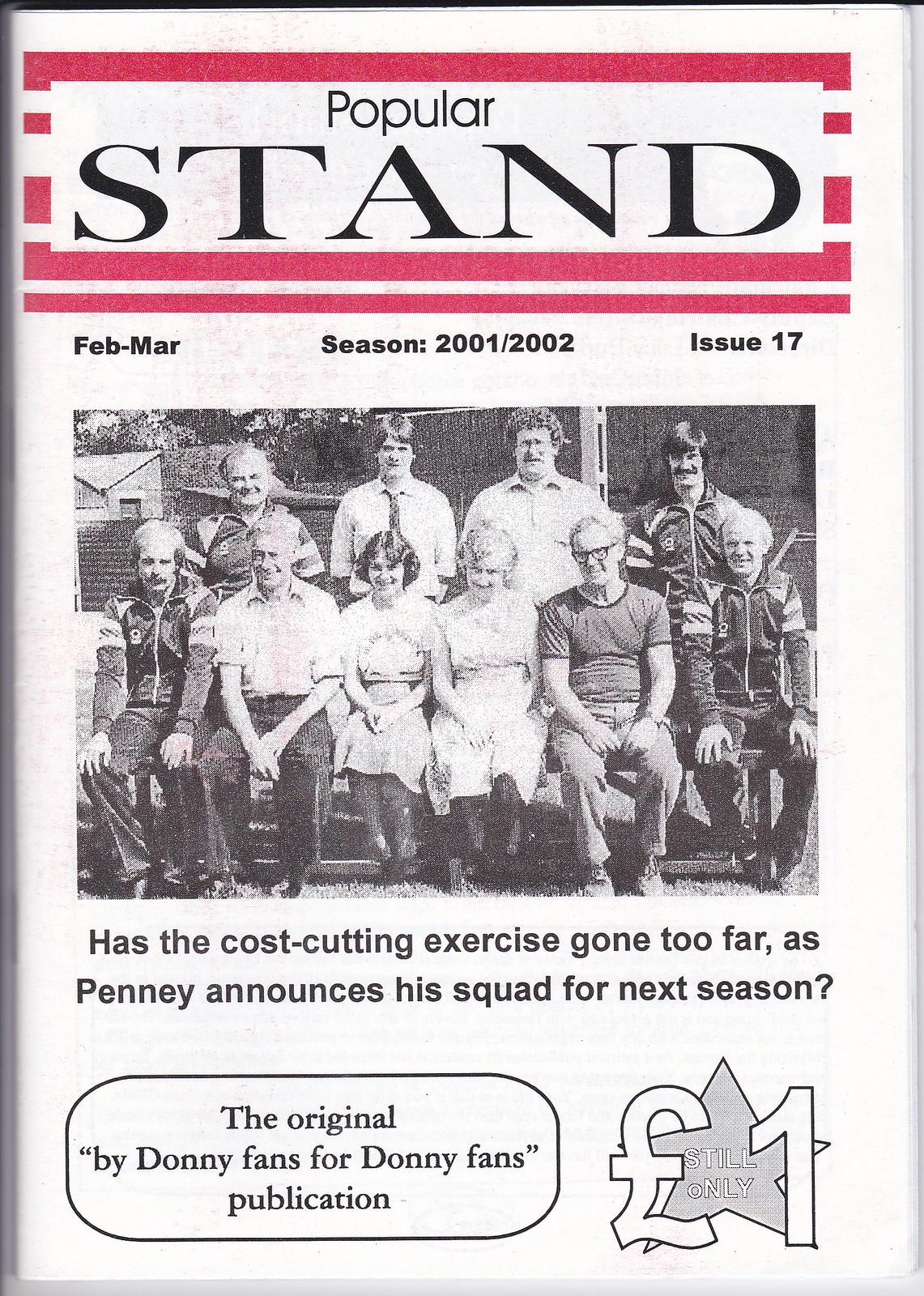The front page of the European magazine "Popular Stand" from the February-March season of 2001-2002, Issue 17, is framed by a striking red border and features the title prominently displayed with the word "Stand" in bold, capital letters. The background is primarily white, and the top section features two red stripes. Below the title, there is a significant black-and-white group photo of approximately ten individuals, likely from the 1960s or 1970s, sitting and standing on bleachers with houses visible in the distance. They appear to be in their 20s and are dressed in various types of clothing. The accompanying headline reads, "Has the cost-cutting exercise gone too far as Penney announces his squad for next season?" with Penney spelled "P N N E Y." Additional text at the bottom states, "The original by Donnie fans for Donnie fans publication," and highlights the price as "still only one dollar in euro/pound."